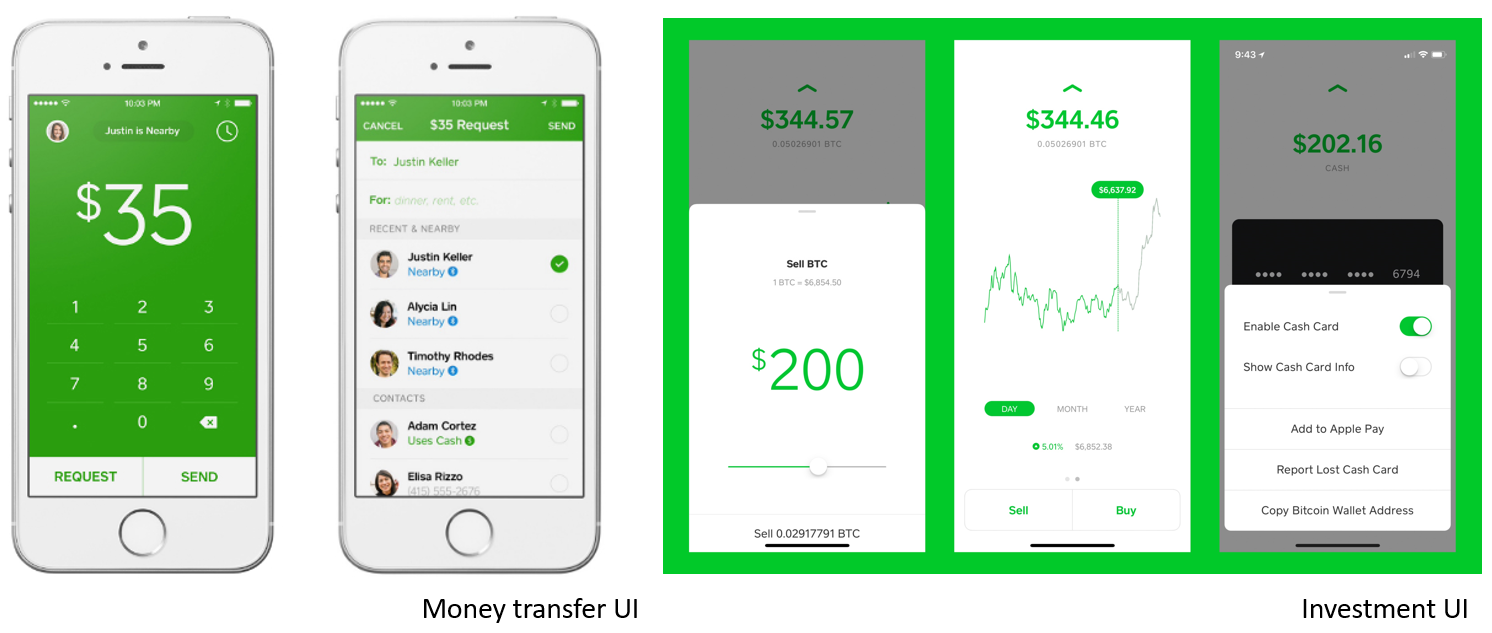This image collage showcases several screenshots from what appears to be a mobile financial application, possibly named "Cash" based on the context and branding.

On the far left, there are two white iPhone SE devices. The leftmost iPhone displays a user interface with a green background displaying "$35" prominently. Above this amount, there's a clock icon flanked by a user picture. Below the amount, a dial pad is visible with digits 1 through 9, an asterisk, zero, and a back button. Two links beneath the dial pad suggest options to "Request" or "Send," indicating a money transfer feature similar to Venmo or PayPal.

The second iPhone screenshot to its right details a screen where a user can request or send $35. The top-left corner shows a "Cancel" option. Below it, the "To" address field is populated with "Justin Keller," and there's a "For" input field that's customizable. The screen lists contacts categorized as "Recent" or "Nearby," highlighting users like Justin Keller (checked), Alicia Lin, and Timothy Rhodes, all tagged as nearby. Additional contacts include Adam Kordex and Elsa Rizzo, with Adam noted as also using "Cash." The app's name, "Cash," is displayed in green letters under Adam's name.

To the right of these iPhones, against a green background, are three additional screenshots. The first one shows a balance of "$344.57" with an option to sell Bitcoin (BTC) for $200. The middle screenshot shows a balance of "$344.46" along with a line graph tracking financial performance. The rightmost screenshot indicates a balance of "$202.16" and features options related to a Cash Card. The "Enable Cash Card" toggle is on, while "Show Cash Card Info" is off. Additional options include "Add to Apple Pay," "Report lost Cash Card," and "Copy Bitcoin wallet address."

Text on the bottom of the image provides UI labels: "money transfer UI" for the two iPhones on the left, and "investment UI" for the three screenshots on the right.